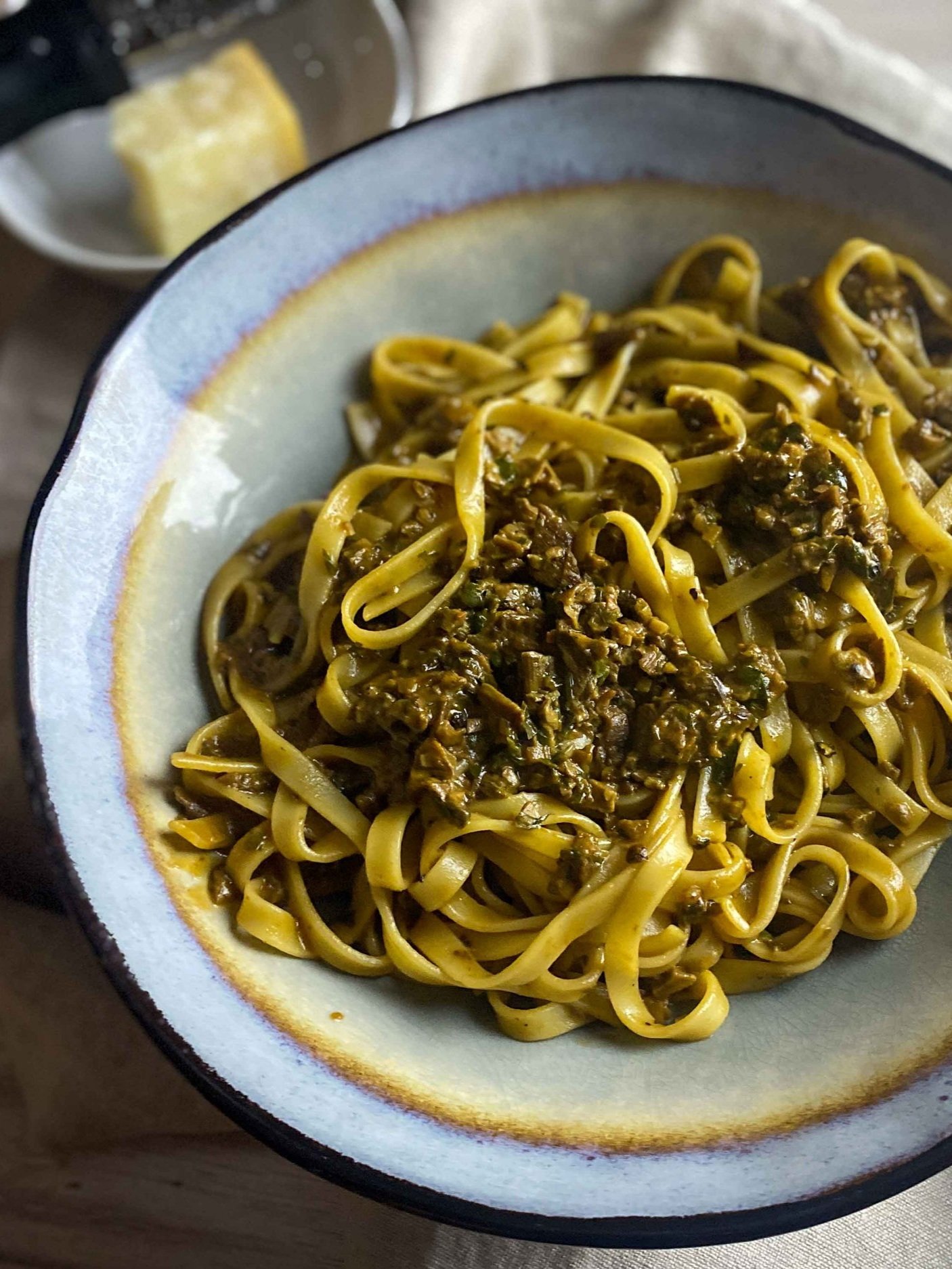The close-up photo captures a hearty bowl of golden-yellow egg noodles, resembling fettuccine or linguine, that glisten with a light oil coating. The pasta is topped with a rich, dark brown meat sauce made of finely shredded beef, and garnished with green herbs, likely oregano, which adds an aromatic touch. The bowl itself is a noteworthy ceramic piece with a somewhat misshapen, handmade quality, featuring an outer rim with shades of brown, a vivid blue inner border, and a gradient fading to light yellow. Perched on a wooden table, or possibly an off-white, textured tablecloth, the scene is complemented by a small, gray bowl in the upper left corner that holds a chunk of light yellow Parmesan cheese, with a black grater resting over it.